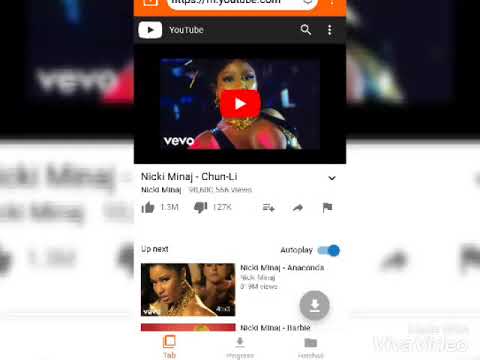The image depicts a YouTube video of Nicki Minaj playing on a screen. The interface appears to be an overlay superimposed on the background, showing various details of the YouTube page. At the top of the overlay, there is an orange URL bar displaying the YouTube link, with a magnifying glass and a horizontal dot menu on the top right corner. 

The video currently shown is Nicki Minaj's "Chun-Li." Just below the video title, there is a like button with 1.1 million likes and a dislike button with 127K dislikes. The interface also includes options for adding to a playlist, sharing, and flagging the video. 

To the right, there is a list of suggested videos under the "Up next" section, with autoplay toggled on, indicated by a blue bar. The top video in this list is "Anaconda" by Nicki Minaj, which has garnered 2.9 million views. The thumbnail image of the suggested video is displayed to the left of the video title.